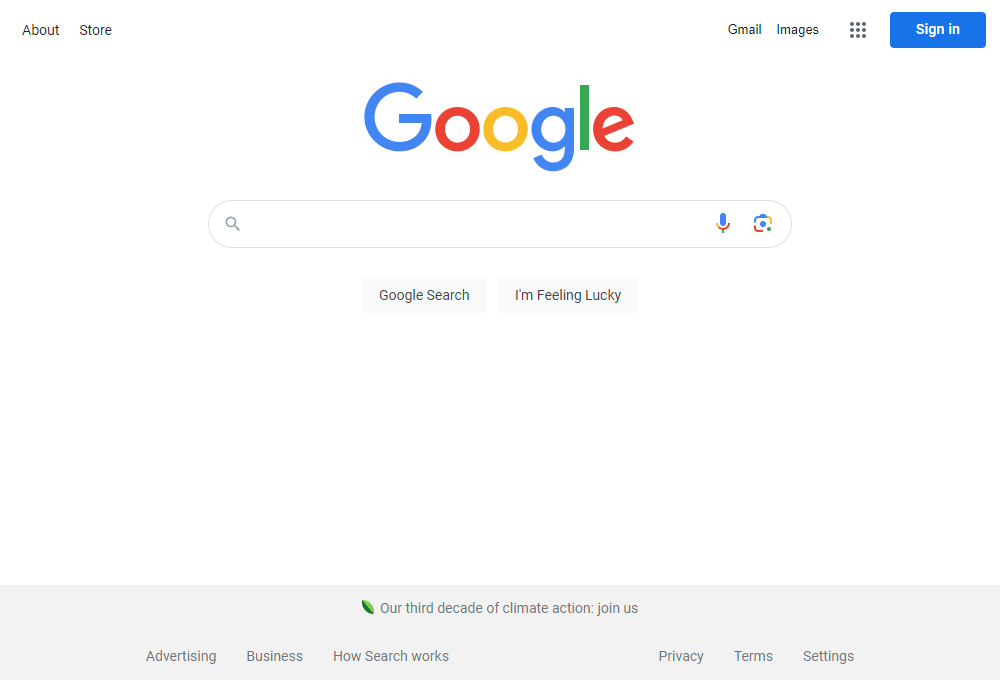This image depicts the Google search homepage. The layout is structured with several elements aligned horizontally along the top of the page. 

In the upper left-hand corner, the word "About" is displayed in black font with a capital 'A'. Following it is a spaced gap, leading to the word "Store" in the same black font and of identical size with a capital 'S'. There are multiple spaces after "Store," which then lead to the right side where additional elements reside.

On the right side, also aligned horizontally, we see "Gmail" with a capital 'G' in the same black font, followed by a space. Next comes the word "Images," again in black font with a capital 'I'. Adjacent to "Images," there is an icon depicting a square made up of smaller circles. Following this is a space, succeeded by a "Sign In" button.

Centrally positioned below these elements is the word "Google" displayed prominently. Below "Google" is a significant space, leading to the focal point of the page— the Google search bar, which is centrally aligned and inviting users to input their search queries.